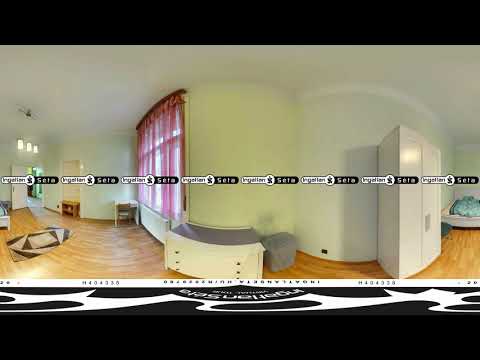The photograph depicts the interior of a room with a blend of different elements. The walls exhibit a mix of yellow and white tones with a predominant yellow hue on the left and white on the right. Central to the room is a white dresser adorned with gold handles, a grey or blue item on top, and flanked by a grey stool or bin. Right of this dresser is a larger, vertical white wardrobe. A rectangular carpet with a beige and brown pattern is positioned on the left side of the light brown wooden floor, along with a patterned black and white area rug featuring a sequence of rotated squares.

The window, centrally located, is complemented by sheer pink curtains. Three wall-mounted lights in a row are situated on the left side near the open, white door, which provides a glimpse into the adjacent space. A white fan is installed on the ceiling, positioned near the three wall lights. A bed, visible on the right, has a white frame with a blue cover.

Overlaying the entire image are bands of black and white with some text, partially unreadable, and circular logos, adding further layers of visual complexity.